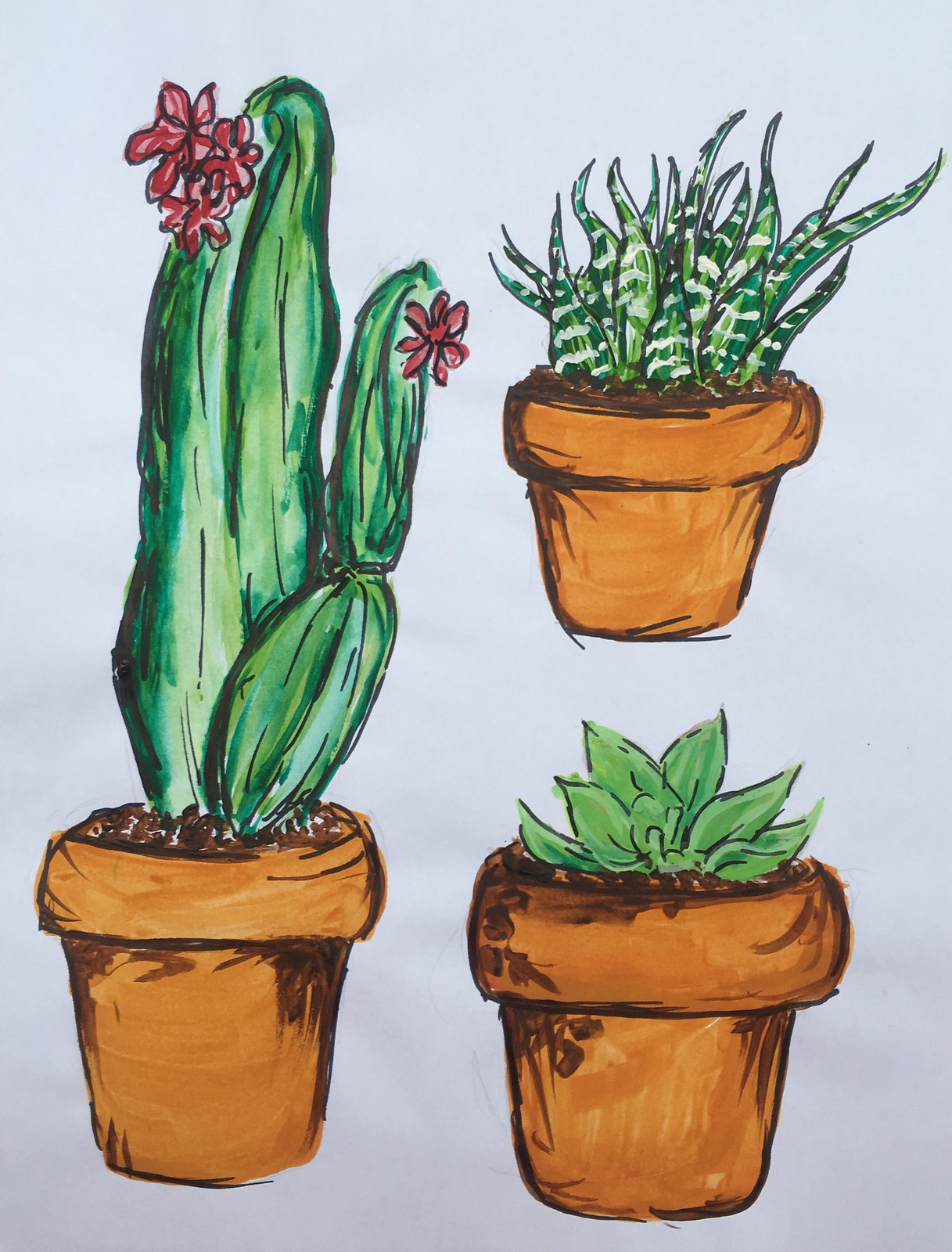This artwork beautifully captures an assortment of potted plants, meticulously drawn with pencil and subsequently enhanced with vibrant colors. The central focus is on three distinct plant illustrations, each housed in similar clay pots characterized by a warm orangish-yellow hue accented with brown tones. The tallest of the trio is a green cactus with subtle yellow accents, thriving in an earthy brown soil. It features several pink blossoms crowning its top and adorning its sides, adding a striking contrast to the cactus's spiny texture. Adjacent to the cactus is a depiction of a spider plant, notable for its shorter stature and distinctive green leaves adorned with white stripes. The third plant, depicted at the bottom, showcases smooth, lush green leaves that unfurl gracefully from its pot. This detailed rendering showcases the artist's exceptional skill in blending different mediums to create a lively and realistic portrayal of potted plants.